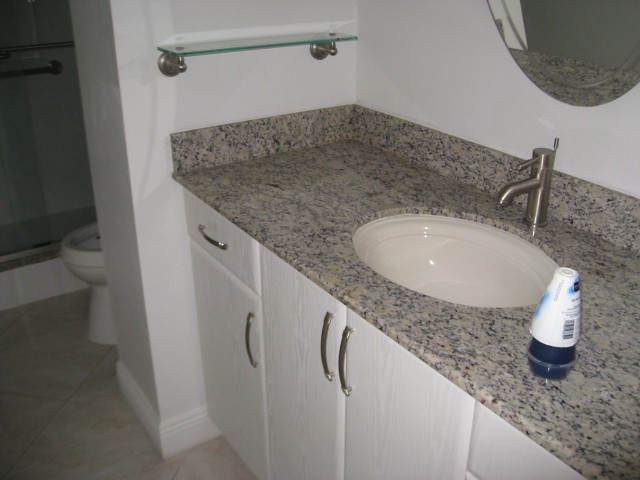This photo showcases a pristine single-sink bathroom. The elegant countertop, crafted from white granite with black speckles, features a 1-2 inch matching backsplash that encircles its perimeter. Positioned next to the sleek sink faucet, finished in pewter, sits a triangular-shaped air freshener with a pop-up lid. An oval mirror is mounted on the white-painted wall above the sink. To the left, a glass shelf with silver mounting brackets provides an additional storage option. The lower cabinet, displaying a subtle wood grain pattern, is painted white and adorned with silver strip-style knobs; the horizontal pull on the drawer contrasts with the vertical pulls on the cabinet doors. The floor is finished with large, elegant marble tiles, adding to the sophisticated aesthetic. A glimpse of the toilet, featuring its lid up, can be seen peeking into the scene.